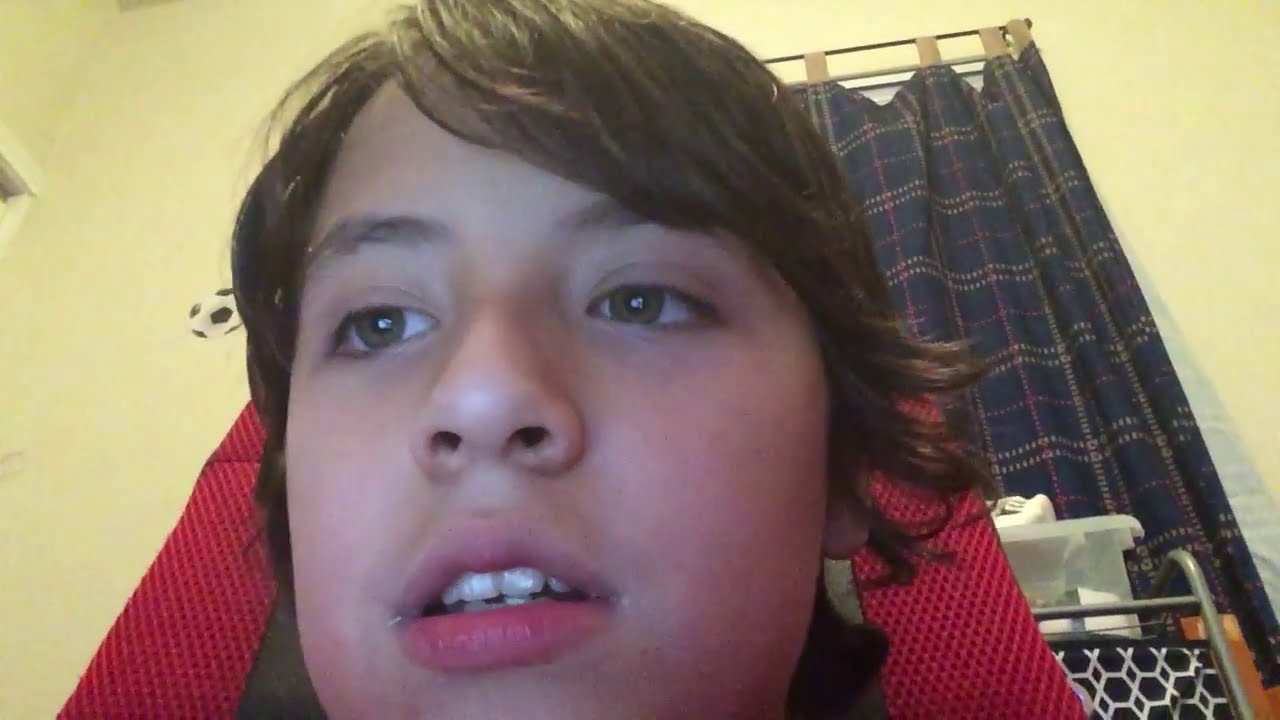This highly detailed close-up photograph captures a young boy, around 10 to 14 years old, with Caucasian features. He has brown hair, parted to the left and slightly shaggy, with some curls near his ears. His hazel eyes, a mix of greenish-brown, are focused slightly to his right, possibly at a computer screen, giving him a thoughtful expression. His mouth is slightly open, revealing his top four teeth, and a hint of his lower teeth.

The boy is seated in a red chair, which is prominently visible in the image. Behind him, the indoor setting features a yellow wall adorned with a small, decal-style soccer ball sticker. To the right, a blue plaid curtain with red and white stripes hangs over a window. Additionally, in the background, one can faintly see a rack with a tub on it and a hexagonal black and white design underneath.

Overall, the image provides a rich, domestic scene, capturing the boy in a moment of quiet concentration within his familiar surroundings.